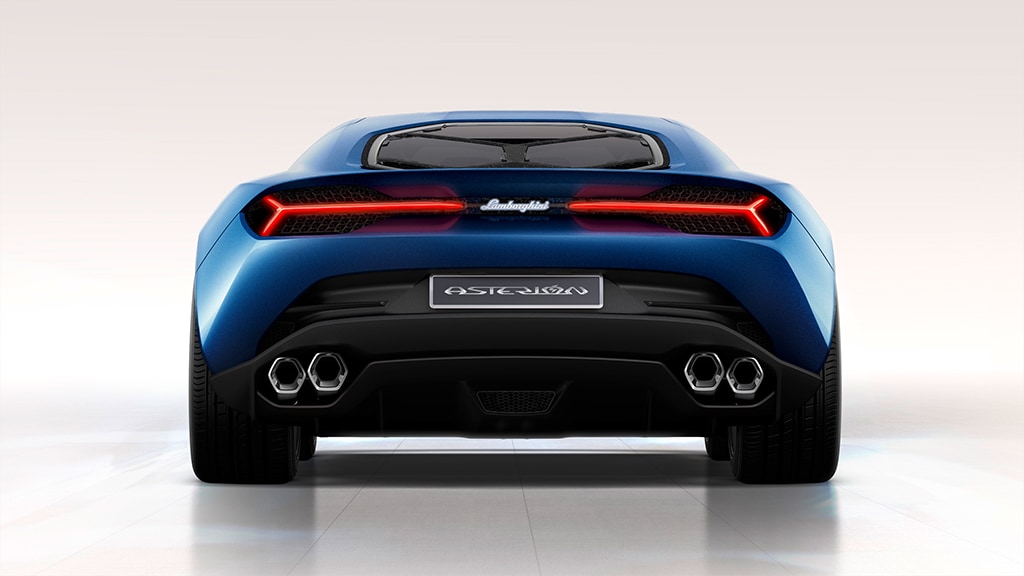This image showcases a highly detailed, likely computer-rendered, rear view of a blue Lamborghini Asterion sports car, framed against a gray-pink wall and resting on a white-tiled floor. The car's slick, aerodynamic design is accentuated by its streamlined black bumper and wide, black racing-style tires. Central to the composition, the brand name "Lamborghini" is prominently displayed in white lettering between the elongated taillights, which feature red linear styling with outward flaring ends. The car's sleek profile includes a tinted, smallish oval rear window and a matching blue roof. Notable details include the double tailpipes on each side, the molded black bumper, and the reflective surface beneath the car, which curiously only mirrors the tires. The large, rectangular license plate reads "ASTERION," completing the detailed rear view of this captivating vehicle.